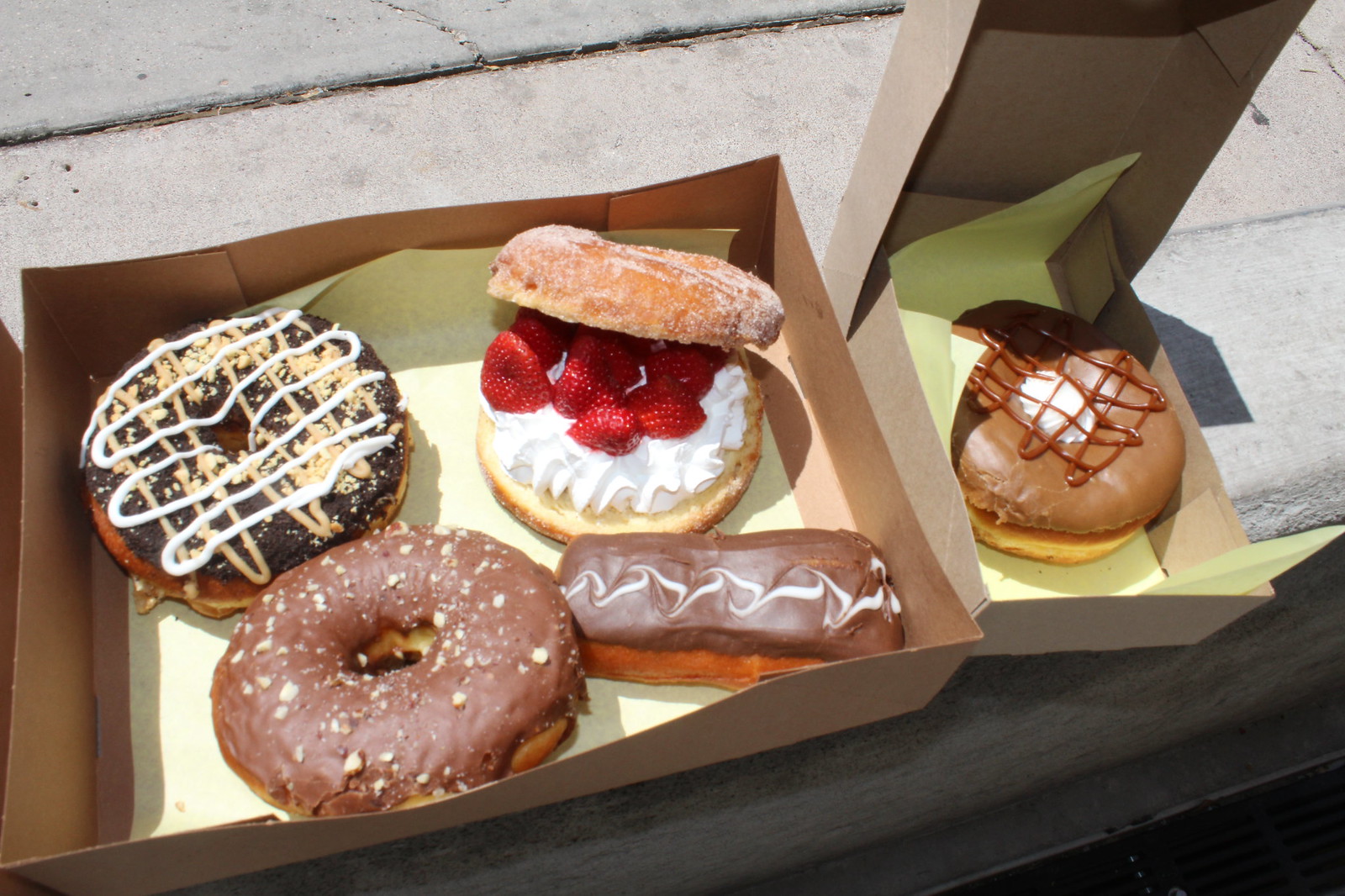In this photograph, we see two cardboard boxes of assorted doughnuts resting on a gray concrete curb, against a backdrop of sidewalk slabs with dirt in between. The larger, lidless box on the left contains four different doughnuts neatly arranged. In the upper left corner, there is a dark chocolate frosted doughnut with intricate swirls of white and tan frosting, possibly accented with nuts. Below it, in the lower left corner, lies another chocolate glazed doughnut, this one adorned with crumbles. Occupying the lower right corner is a long, rectangular chocolate-covered eclair with a delicate white drizzle. The upper right corner features a unique doughnut that has been sliced in half to reveal a filling of whipped cream and fresh strawberries, with a sugary exterior. To the right of this large box is a smaller box with its lid open, showcasing a single doughnut. This doughnut appears to be a Boston cream with a smooth chocolate glaze and a decorative chocolate drizzle. The vivid details of the doughnuts, coupled with the casual placement on the concrete curb, suggest a relaxed, impromptu treat awaiting someone to enjoy.